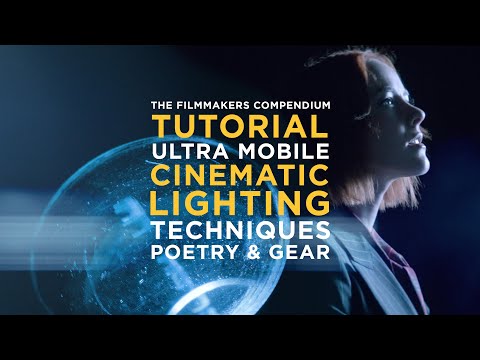The image is a dark, computer-generated depiction of a woman with straight, shoulder-length red hair and a suit jacket with lapels. She is looking off to the right, and her face is illuminated by a blue light, creating a distinctive hue. The background features a translucent, jellyfish-like object or clear glass globe behind her. Overlaying the image are the words "The Filmmaker's Compendium Tutorial: Ultramobile Cinematic Lighting Techniques, Poetry, and Gear," suggesting it may be the first slide of a PowerPoint presentation or an advertisement. Thick black borders frame the top and bottom of the picture.